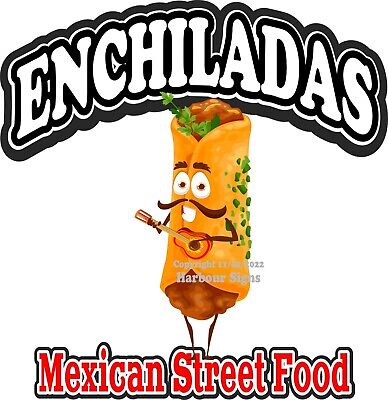The image is a digital advertisement for Mexican street food featuring a whimsical, personified enchilada against a pure white background. The top text reads "ENCHILADAS" in bold, white capital letters outlined in black, while the bottom text states "Mexican street food" in red, also outlined in black. In the center, there is a character resembling an enchilada with a smiling face, featuring expressive brown eyebrows, white eyes with black dots, a curved mustache, and white teeth. This enchilada character is playfully decorated with cilantro and refried beans forming its body and hair, and it has small arms and spindly legs. The figure is holding an orange and yellow guitar across its belly, adding to its cheerful demeanor. On the right side of its body and near the top, there are green specks, possibly parsley or cilantro, enhancing the design. The bottom of the character has a text line containing copyright information, indicating it is © 2022 Harbor Signs.